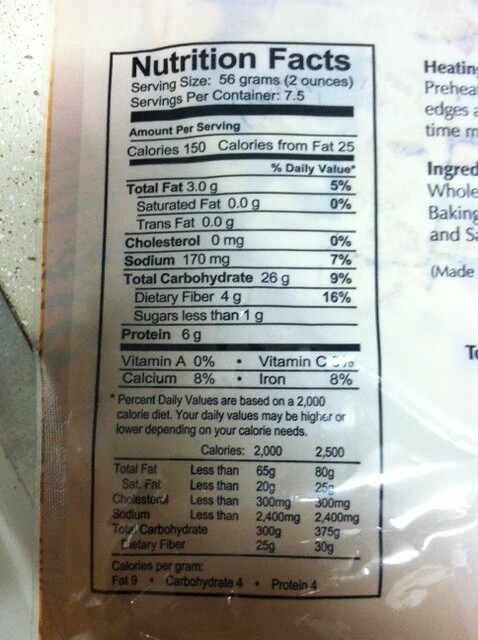This is an indoor, close-up color photograph of the left side of the back of a clear plastic package, positioned on a white laminated countertop with black and white speckles. The image prominently features a Nutrition Facts label, which is bordered in black. The package reflects some light from above, highlighting its clear nature. The Nutrition Facts label starts with "Nutrition Facts" at the top and details a serving size of 56 grams (2 ounces) and 7.5 servings per container. Each serving provides 150 calories, with 25 calories from fat. It lists various nutritional details including total fat (3 grams), cholesterol (0), sodium, total carbohydrates (26 grams), dietary fiber, sugars, and protein (6 grams). The label also includes vitamin levels, specifically noting 8% for both calcium and iron. At the very bottom, it mentions the calorie values per gram: fat (9), carbohydrate (4), and protein (4). The label indicates that the percent daily values are based on a 2,000 calorie diet and cautions that individual daily values may vary. Partially visible at the top right corner of the image, cut off by the edge, are the heating instructions and the ingredients list.